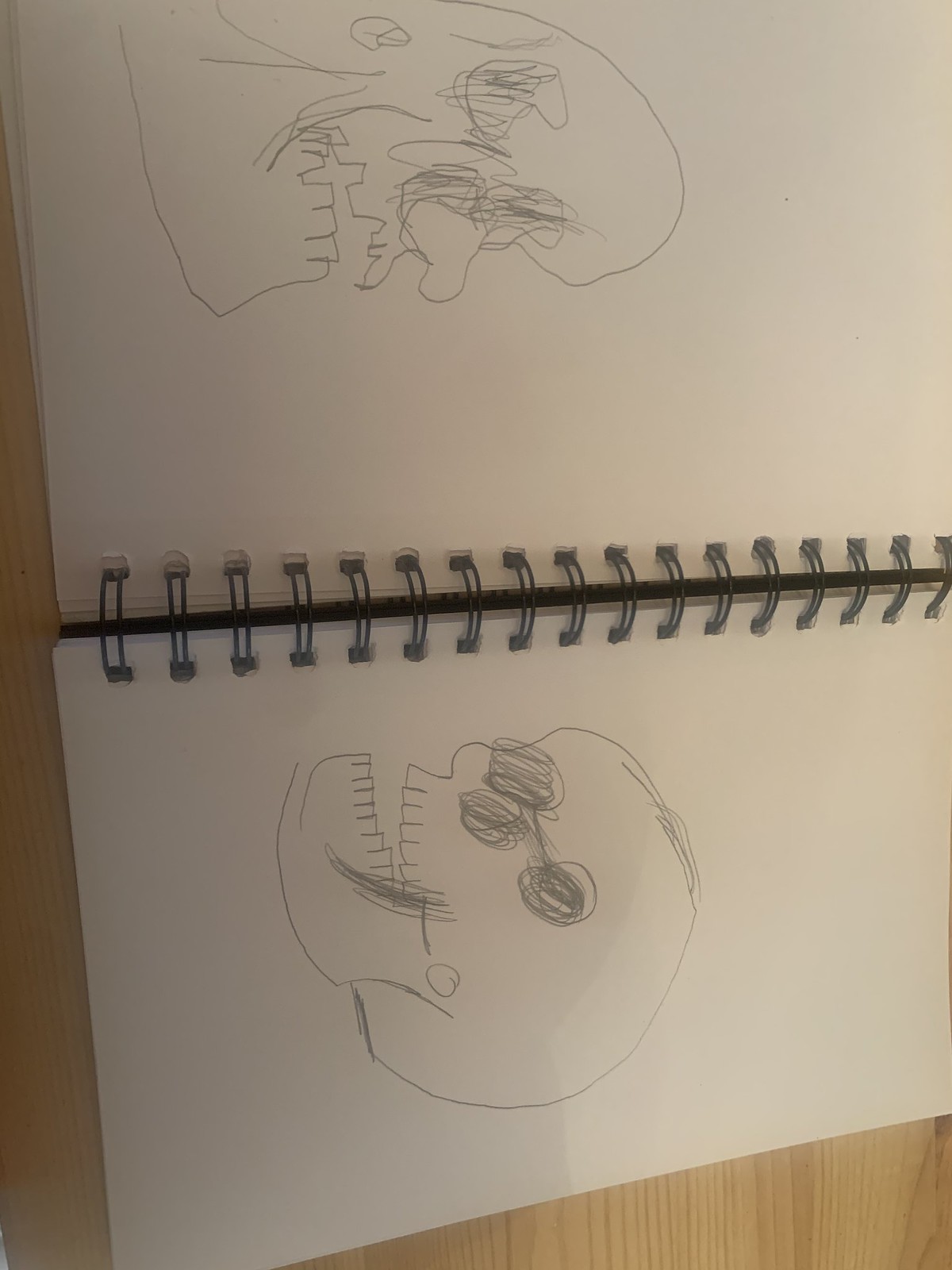This photograph captures an open, spiral-bound sketchbook lying on a light-colored wooden table, oriented horizontally with the spine running across the middle. The sketchbook is rotated 90 degrees to the right, making the left page appear at the top of the image and the right page at the bottom. The black metal binder divides the white pages, which feature two rudimentary pencil sketches of skulls. 

The top page showcases a right-facing skull profile with a large, exaggerated nose, craggy teeth, and dark, scratchy eyes. The chin is quite square, and the overall features resemble a Pac-Man ghost, suggesting a child-like simplicity in the drawing.

The bottom page contains a left-facing skull with a more traditional look. This skull has straight teeth, dark eye sockets, and an identifiable hinge at the jaw. Both drawings exhibit a crude, simplistic style that adds to their slightly eerie charm.